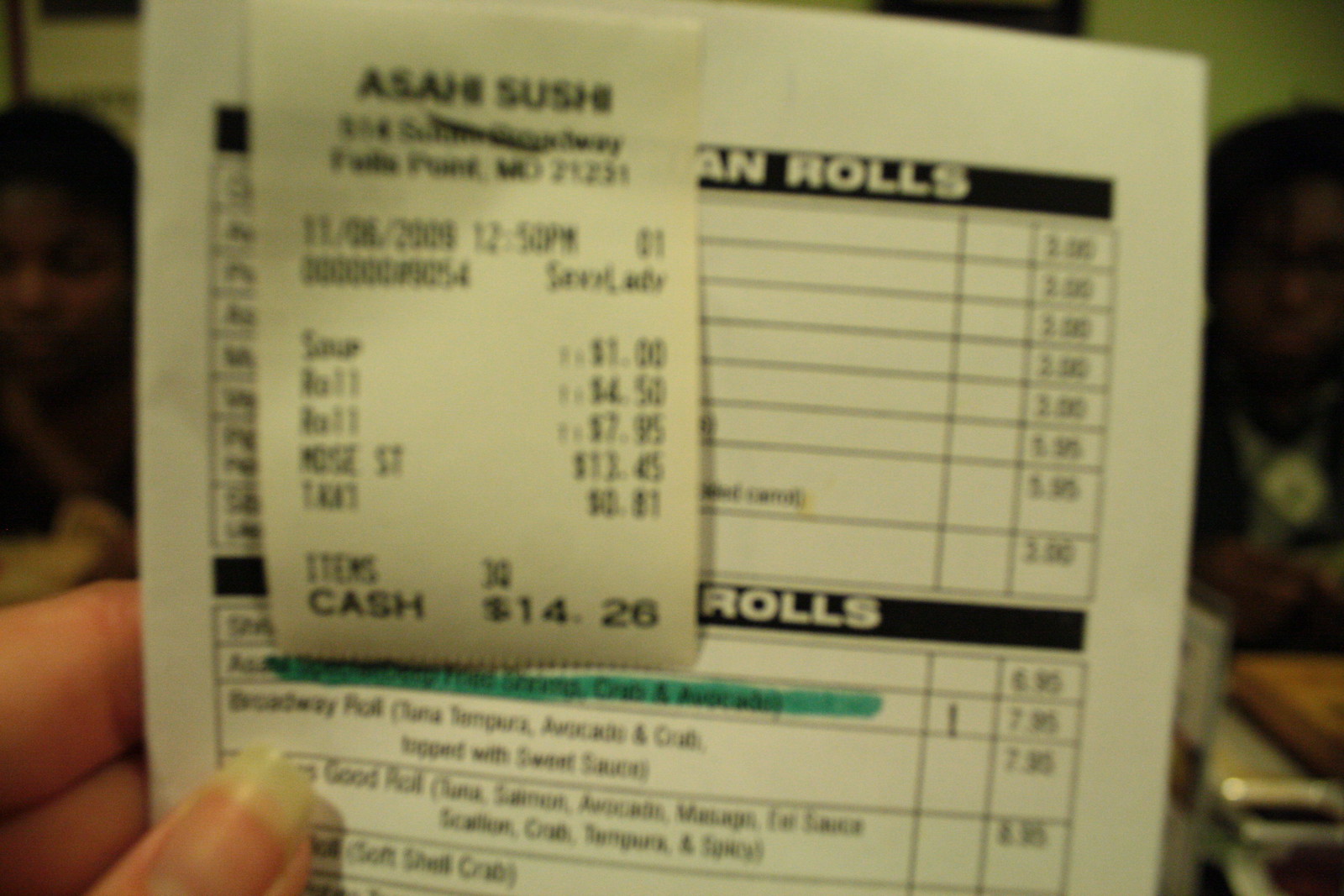In the photograph, a person's left hand prominently displays a receipt, with their thumbnail, index finger, and middle finger clearly visible. The receipt is relatively small and has a menu stapled to its length. The establishment's name, "ASAJ's Sushi," is legible at the top of the receipt. Although the address on the receipt is blurry and difficult to discern, the date stamp indicates the transaction took place on November 6, 2006, at 12:50 p.m. The total amount spent is recorded as $14.26. Notably, an item on the menu, priced at $2.95, is highlighted in green, drawing immediate attention. The photo captures the detailed textures of the receipt paper and the crispness of the highlighted menu item, adding depth to the overall composition.